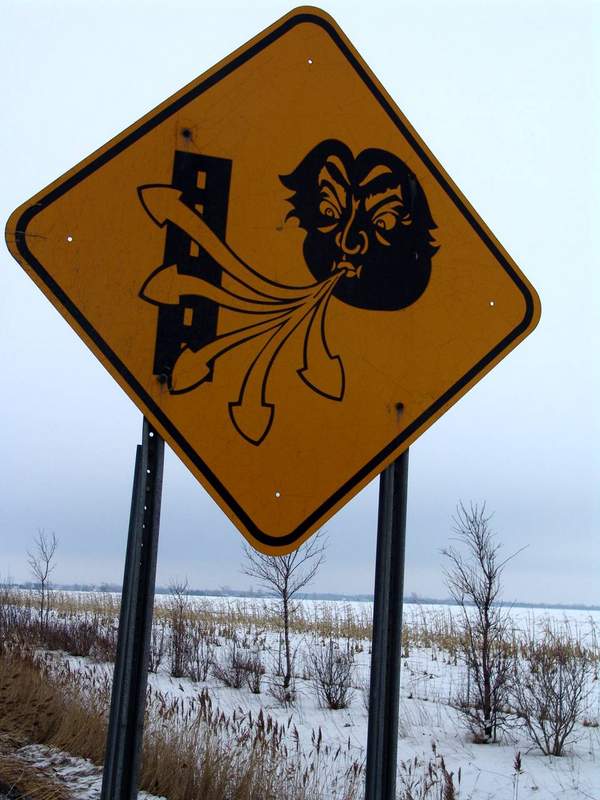A humorous photograph captures a diamond-shaped, orange traffic sign on a snowy freeway. The sign, outlined with a black border, warns of extreme wind conditions with a quirky illustration. A tall building, depicted with a small maze-like structure on top that initially resembles a spiderweb, is actually part of the rusted net securing the sign to two holding poles. The amusing centerpiece of the sign features a giant face, personifying the wind, blowing five arrows of gust towards the towering building as if it's about to topple. The wind face is depicted with an exaggerated look of determination and anger. In the background, the landscape is covered in snow, with sparse brown plants dotting the ground, and the sky appears foggy and white, enhancing the wintry scene.